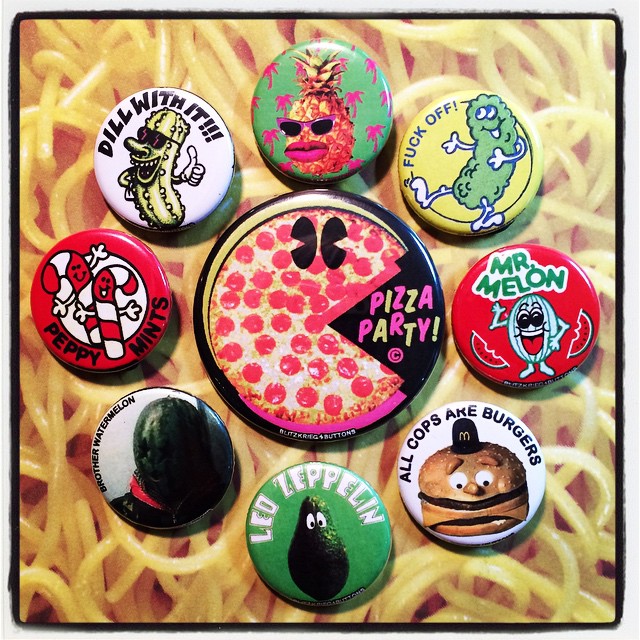The image showcases a vibrant collection of 10 whimsical pins, artfully displayed against a spaghetti background. At the center, a large pin features a pepperoni pizza designed to resemble Pac-Man, with a missing slice and the words "Pizza Party" inscribed. Surrounding this centerpiece are nine smaller, cartoon-like pins, each with its quirky design: 

- A pineapple character with sunglasses, pink lipstick, and palm trees in the background.
- A dill pickle with the message "Deal with it," wearing glasses and smiling.
- A red pin labeled "Peppy Mints," depicting two peppermint sticks.
- A pin showing a watermelon, titled "Brother Watermelon."
- An avocado with the amusing caption, "Let that guac."
- A hamburger with eyes and a nose, donning a McDonald's hat, and the phrase "All cops are burgers."
- A green pickle with the profane message "Fuck off."
- A red pin with the title "Mr. Melon," showcasing a cartoon-like melon character.

This eclectic mix of pins creates a playful and colorful display, each one adding its distinct flair to the pizza-themed centerpiece.